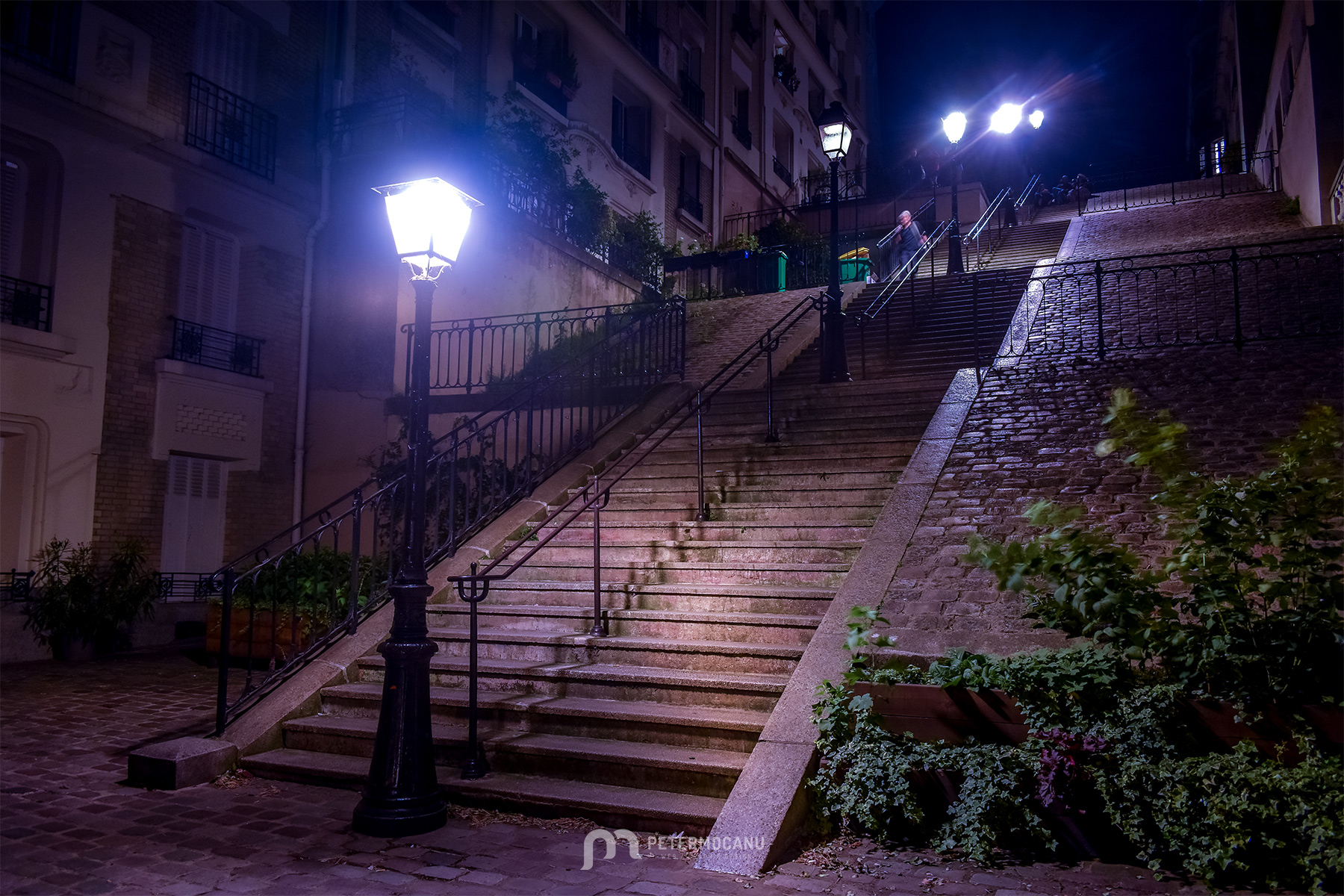In the upper right-hand corner of the image, the dark sky suggests that it is either nighttime or the early hours of the morning. The lower right-hand side features lush green bushes, adding a touch of nature to the scene. Above the bushes, there is a wall made of grayish bricks, which appears solid and structured. Centrally located in the image are a set of stairs, with a dividing pole separating the up and down pathways. Multiple black lamp posts with white tops line the middle of the stairs, casting light on the steps below. A blurry figure is seen descending the stairs, adding a mysterious, dynamic element to the scene. On the left side, a beige and white brick building with barred windows is visible. The bars over the windows likely serve a protective function.